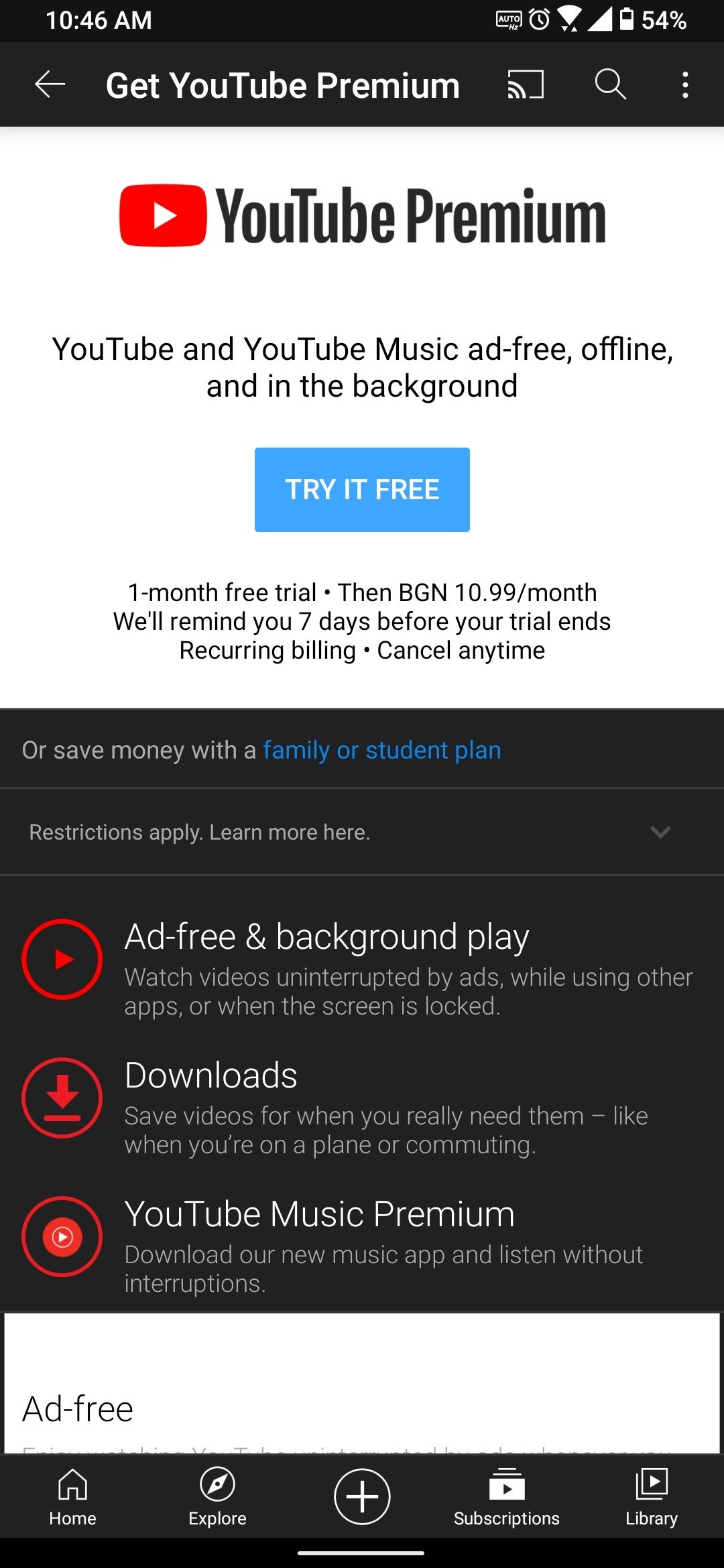Screenshot Description: Promotional Screen for YouTube Premium

The screenshot captures a promotional screen for YouTube Premium, providing a detailed overview of its features and benefits. The screen appears to have been captured at 10:46 AM, as indicated by the time displayed in the top-left corner against a black banner.

On the top right, there is a series of icons: an "Auto" icon in white, followed by an alarm clock icon, a Wi-Fi icon, a signal strength icon, and a battery icon showing 54% charge.

Below this, against a somewhat translucent dark gray background, we observe a left arrow icon next to the text "Get YouTube Premium." Alongside this, there are icons for casting, search (magnifying glass), and a vertical three-dot menu button.

The main section of the screen features a white background with the YouTube logo and the text "YouTube Premium." Underneath, the accompanying text reads, “YouTube and YouTube Music, ad-free, offline, and in the background.” A prominent blue button invites users to "Try it for free," with white text on it. Below this button, black text states, “One month free trial. BGN 10.99/month.” It also mentions, “We’ll remind you seven days before your trial ends. Recurring billing. Cancel anytime.”

Further down, the background returns to black, with text highlighting alternative plans, reading, “Or save money with a family or student plan” in blue and gray text, followed by “Restrictions apply, learn more here” with an arrow indicating more information.

The screen then lists three main features of YouTube Premium with corresponding icons:
1. **Ad-free and background play**: Illustrated with a play button icon and descriptive text explaining uninterrupted video watching while using other apps or when the screen is locked.
2. **Downloads**: Represented by a download icon and text stating you can "save videos for when you really need them" like on a plane or commuting.
3. **YouTube Music Premium**: Denoted by a red circular icon with a play button, and text explaining downloading the music app to listen without interruptions.

Almost at the bottom of the screen, a white banner with black text states "ad-free," though the text below is cut off and not visible.

The bottom navigation icons are also visible, starting from left to right:
- **Home**: Represented by a home icon.
- **Explore**: Represented by a compass icon.
- **Create**: A circle with a plus sign in it.
- **Subscriptions**: Indicated by a YouTube play icon.
- **Library**: A play icon over another play icon indicating library access.

This detailed screenshot provides comprehensive information on the YouTube Premium service and its subscription options.